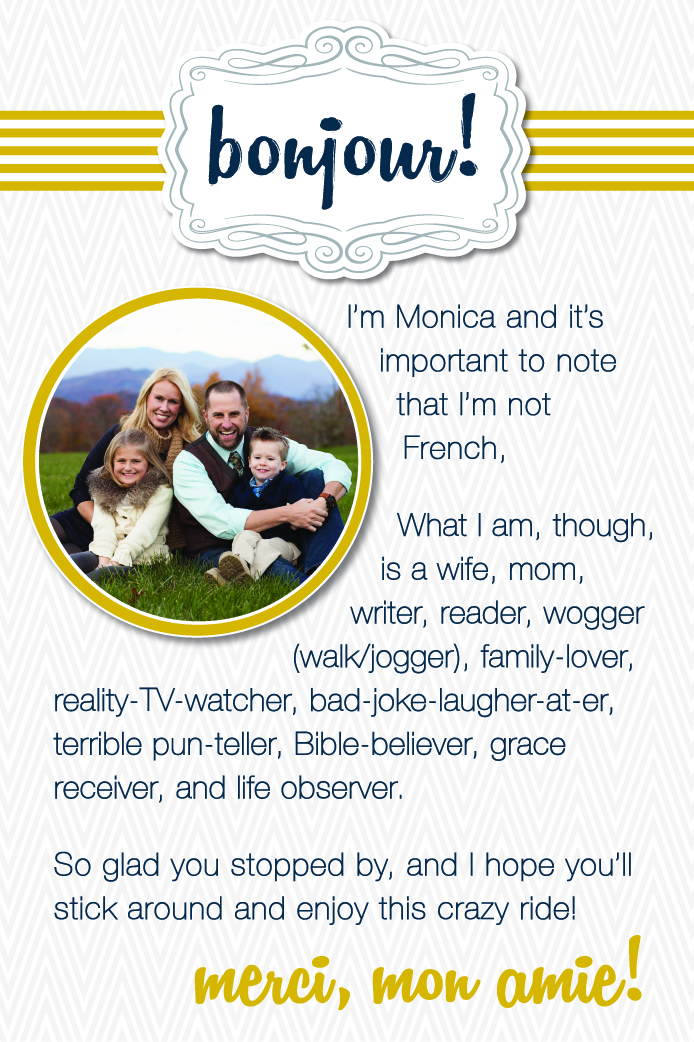This vertical business card-style image features a warm and inviting introduction from Monica. Against a light white and off-gray zigzag-patterned background, it has five gold horizontal bars traversing left to right. At the top, the word "Bonjour" is prominently displayed in a gold-trimmed, black font header. Below this, there's a heartfelt message that reads, "I'm Monica and it's important to note that I'm not French. What I am, though, is a wife, mom, writer, reader, wogger (walk/jogger), family lover, reality TV watcher, bad joke laugher, terrible pun teller, Bible believer, grace receiver, and life observer. So glad you stopped by, and I hope you'll stick around and enjoy this crazy ride."

To the left of this text, a circular photograph bordered in gold showcases Monica's family—herself, with her long blonde hair, her husband in a colored shirt, tie, and vest, their young blonde daughter, and their very young brunette son. The family is seated on grass with a picturesque autumnal backdrop of mountains and trees. This idyllic setting conveys warmth and unity.

At the bottom of the card, in elegant gold cursive, the words "merci, mon ami!" are inscribed, adding a final touch of gratitude and charm.